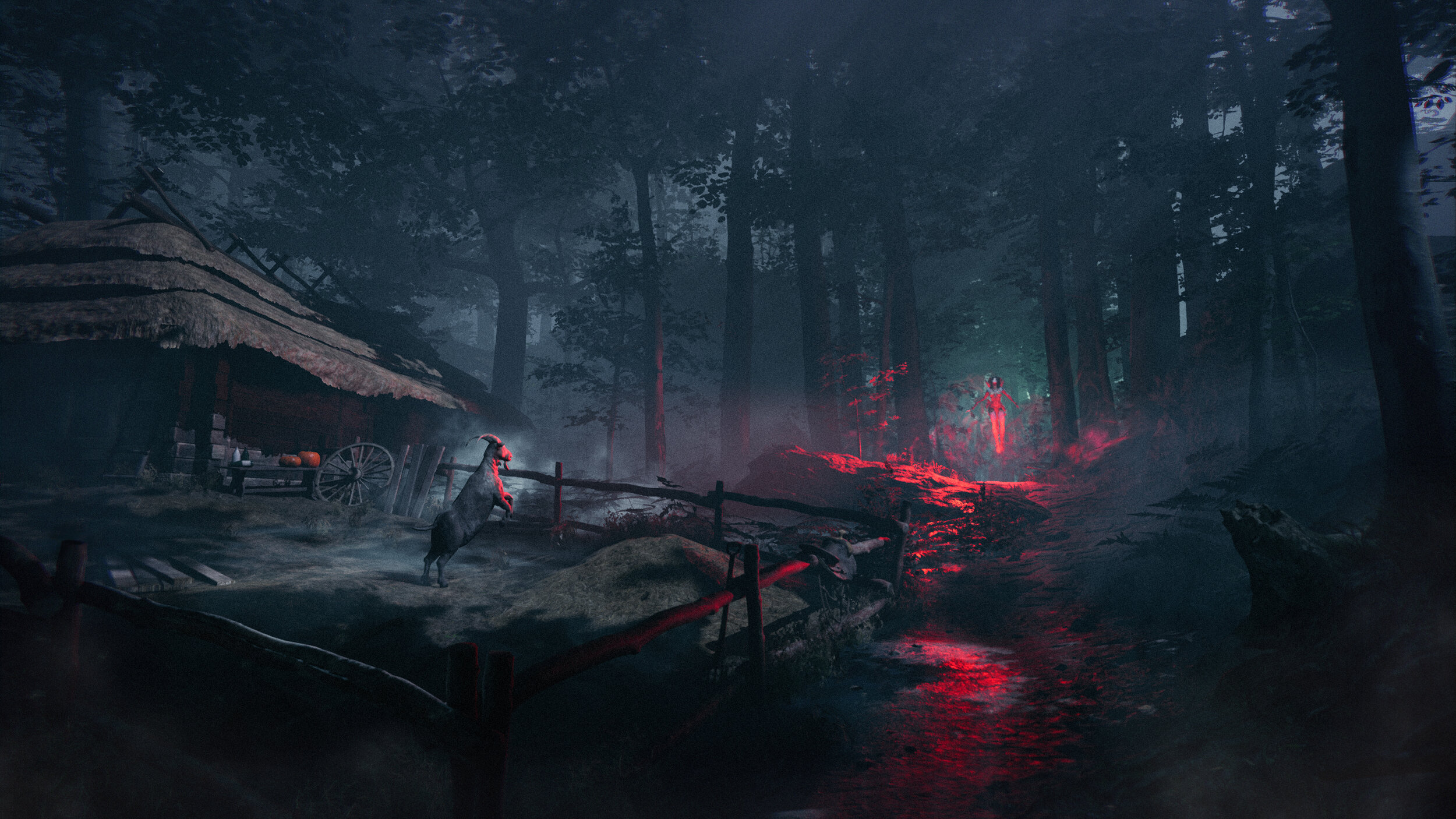The artwork depicts a computer-generated fantasy landscape set during nighttime in a dark forest. The scene features a goat in a pen, rearing up on its hind legs and leaning over a fence. The goat's face has a pinkish hue, enhanced by the illumination from a mysterious, levitating figure. This floating entity, resembling a small person or fairy, emits a radiant red and pink light that casts a glowing aura over the nearby rocks, stream, and the misty surroundings.

To the left of the goat's pen stands a thatched-roof hut, unmistakably a dwelling. The hut is adorned with two pumpkins on a table and a wagon wheel lying on its side by the porch. In the upper left, tall trees with dense foliage frame the scene, with glimpses of a light gray sky and a hill in the distance. The enigmatic floating figure, surrounded by plants, remains the focal point of the composition, adding an air of magic and wonder to the entire landscape.